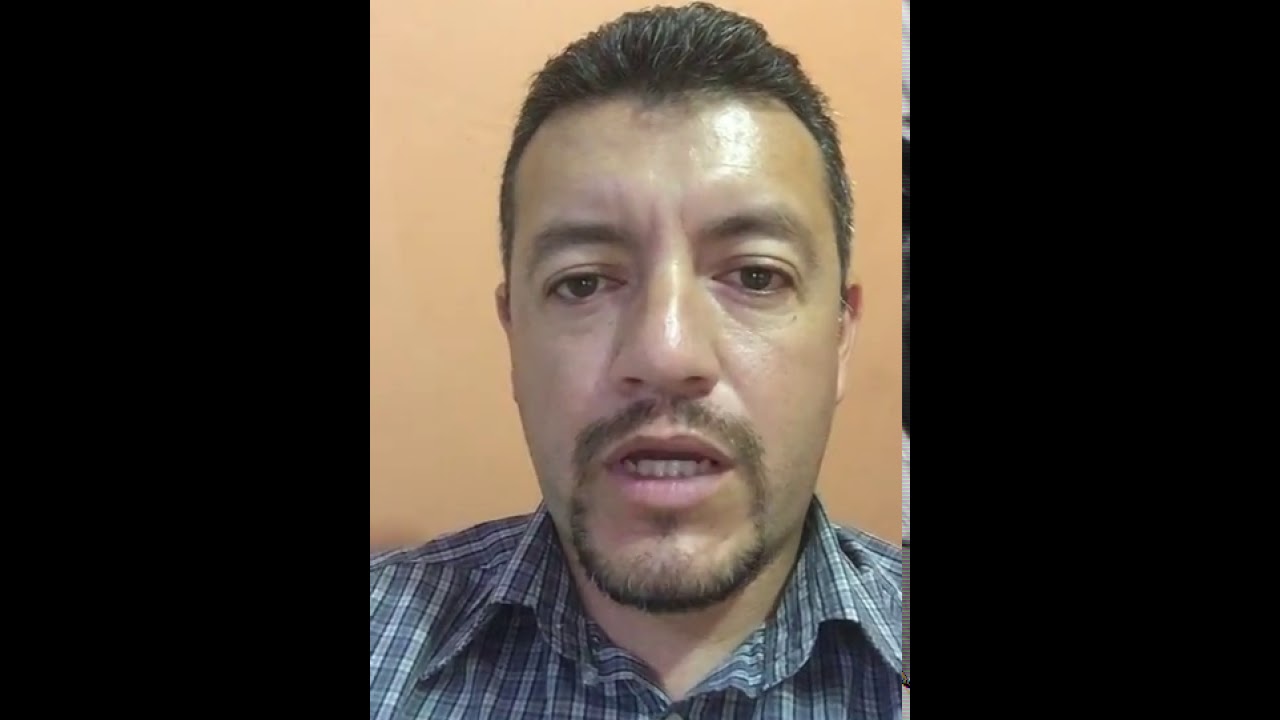This is a close-up photograph of a relatively young man with fair complexion, appearing to be a selfie or a still from a video chat. His face occupies most of the frame and he is looking directly into the camera, apparently in mid-speech, with his mouth open and his lower teeth visible. He has brown eyes, a neatly trimmed goatee, and his short brown hair is closely cropped on the sides and somewhat short on top. He is wearing a greenish check patterned button-up shirt that features a dark to mid-dark green and lighter grayish green checks. The background features a simple peach-colored wall, and there are prominent black borders on both the left and right sides of the image, suggesting the possibility of a screen capture. There is a noticeable glare on his face, particularly on his forehead and the bridge of his nose, indicating that his light source is very close. Overall, the image focuses solely on his facial expression and upper torso, with no additional elements present in the frame.